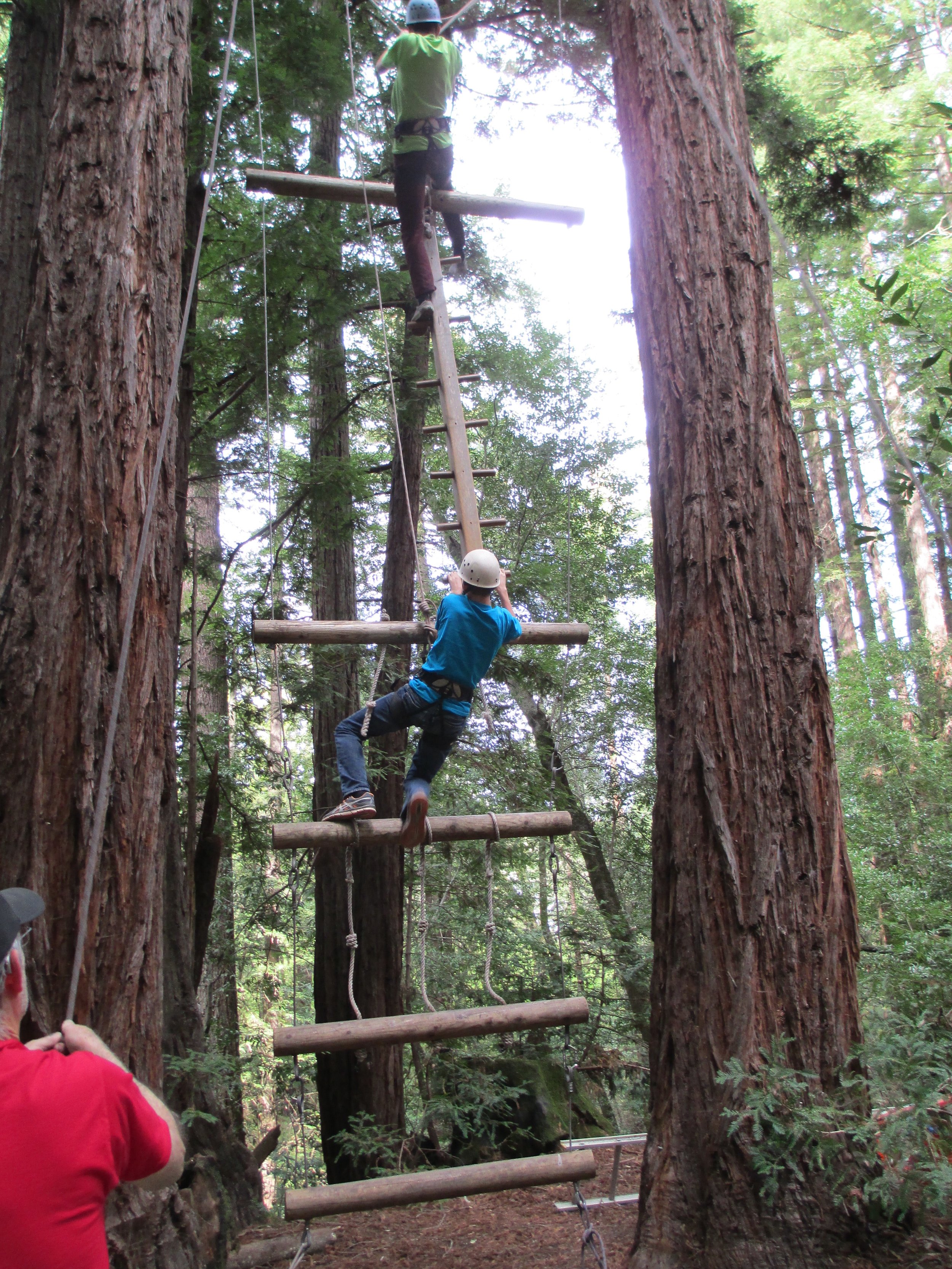In this color photograph, set in a dense forested area, three construction workers are engaged in a tree-climbing task. The image, captured in portrait orientation, prominently features the trunks of two large pine trees on either side. A wooden ladder made of horizontal logs is positioned against the central tree's trunk, forming a makeshift structure for easier ascent. 

One worker, wearing a turquoise t-shirt, cream-colored hardhat, and jeans, is seen climbing this log ladder. He is on the third rung from the bottom and has his hands on a conventional wooden ladder adjacent to the log structure. Near the top of the image, another worker, dressed in a white hardhat, yellow safety vest, and beige pants, straddles the upper section of the wooden ladder, aiding the ascent.

On the ground, below the central tree, stands the third worker. He wears a black visor cap and a red shirt, and is holding a rope attached to the ladder structure, presumably for stability. The background showcases more towering trees and dense forest, emphasizing the workers’ challenging environment. The photograph is a clear representation of realism, capturing the workers in their natural, demanding task within the forest.